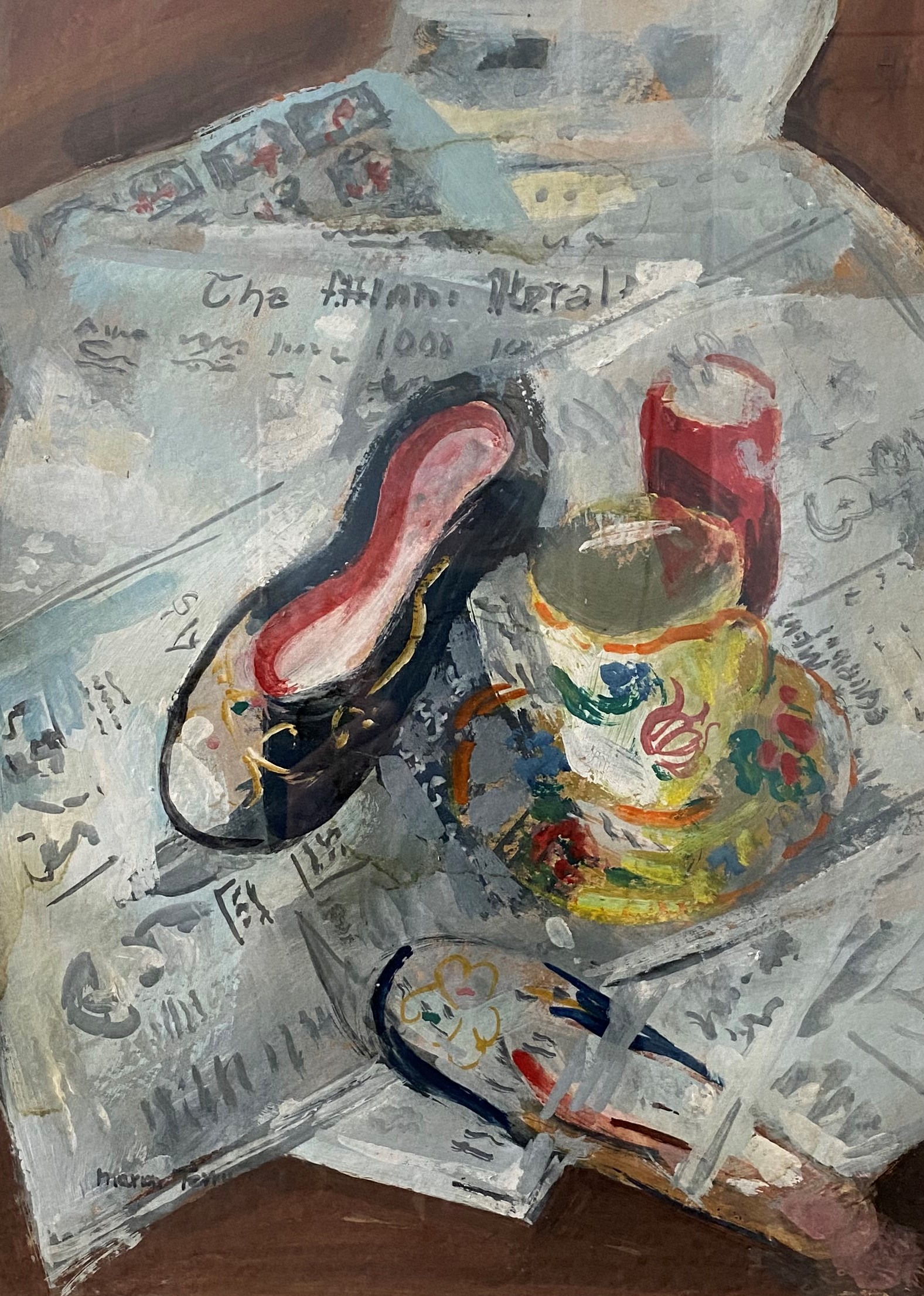The oil painting, in portrait orientation, depicts a cluttered scene with a focus on a stack of newspapers or white advertising sheets, strewn in disarray on a table or surface. The papers, painted in varying shades of light gray with darker gray text and images, are housed within a brown box that contributes to the background. Central to the composition is a black ballet shoe with a red inner lining and various paint smudges—pink near the toe, with gold and yellow lines. To the right of this shoe lies a teacup and saucer adorned in a yellow and white flower pattern, complemented by red, blue, and green spots. A partially visible second shoe, featuring gray overtones as if worn or damaged, is positioned in the bottom right corner. Above this area sits a red can, adding a splash of color to the arrangement. The overall scene employs a smudgy, textured technique, creating a dynamic interplay between the objects and their painted environment.